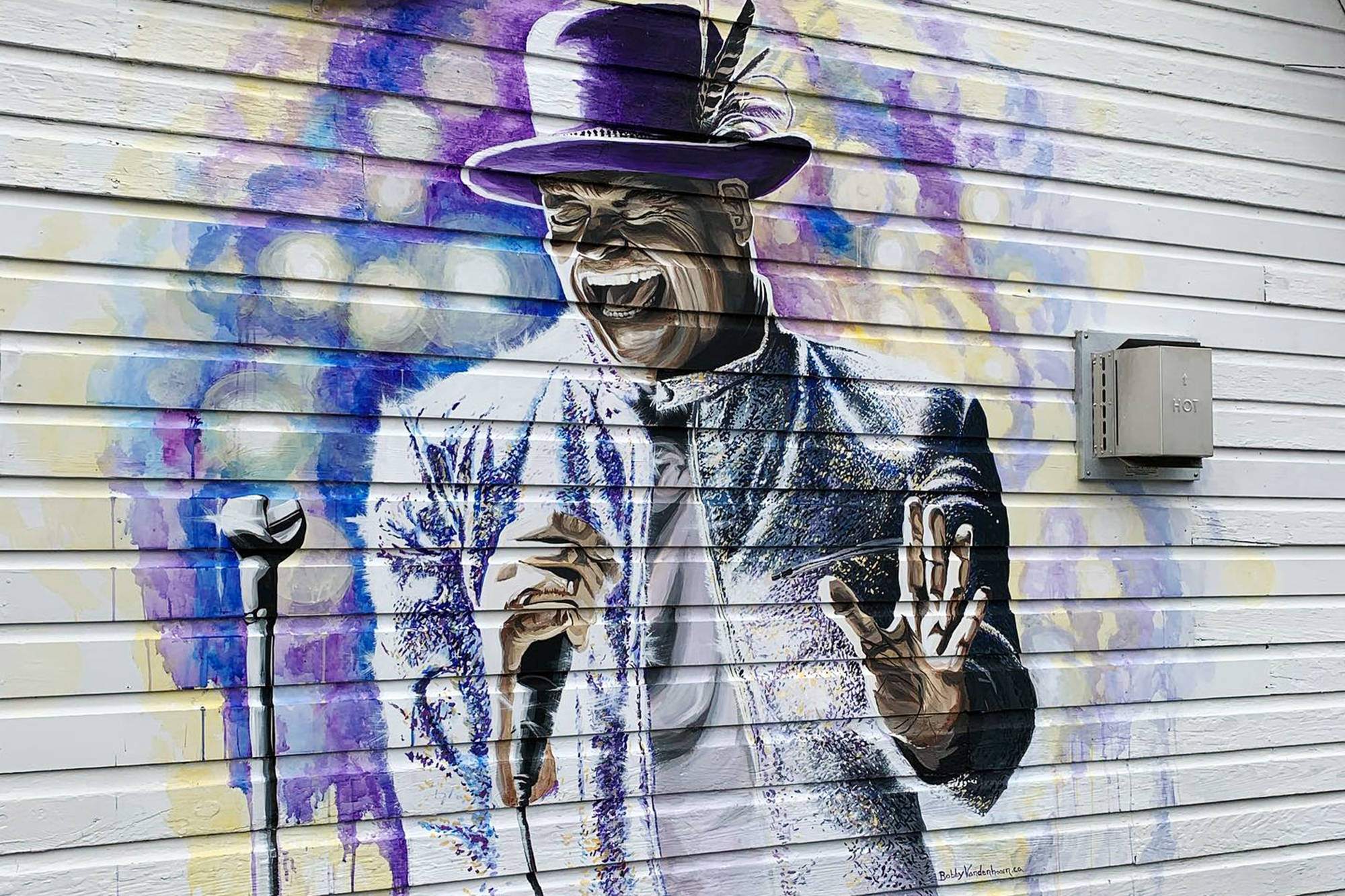This image captures a close-up of a vibrant mural painted on the white siding of a wooden building. It features an African-American man passionately singing into a microphone, his eyes closed and mouth open, caught mid-performance. He is wearing a distinctive mid-length purple top hat adorned with striped black and white feathers on the right side and an additional purple feather at the back. The man's outfit is a striking tuxedo with a gray-purple undershirt; the tuxedo's left side is predominantly white with purple splotches, transitioning to purplish blue on the right, scattered with purple and blue specks, giving it a sparkly appearance. In his left hand, he holds a black microphone, obscured at the top by his fingers, while the right hand is open, expressing his musical fervor. A silver microphone stand stands to his left. The background is an impressionistic blend of vibrant colors, including purple, blue, orange, and yellow, resembling a fireworks display, enhancing the dynamic energy of the scene. To the right of the mural, a gray utility device, likely an air vent, is visible on the wall.